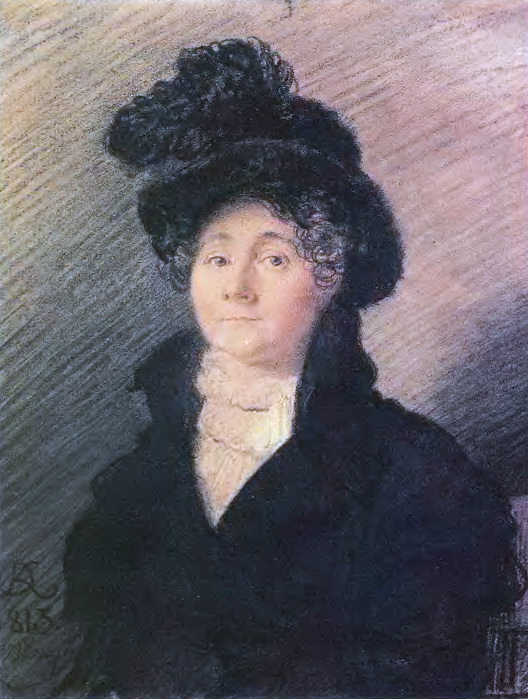This portrait features an older woman, possibly a widow, characterized by her elegant and somber attire. She is clad in a black coat or dress adorned with subtle black ruffles on the arms and a high-standing, ruffled white collar that meets her elaborate, black hat. This formal hat is decorated with black feathers and possibly made of fur, indicating her affluent background. The woman's face, framed by gray curls mostly hidden under her hat, bears a calm, serious expression with a hint of amusement, enhanced by her pale complexion, lovely blue-gray eyes, thin lips, and a broad nose. The background of the painting transitions diagonally from grayish-yellow on the left to pinkish-gray on the right, providing a shadowed yet softly colored backdrop. The portrait is signed with initials and the number "813" in the corner, adding an air of mystery and value to the artwork. Although not explicitly detailed, the hints of a chair edge in the background suggest she might be seated. This painting captures a poised and dignified woman, reflecting her wealth and status through the meticulously detailed and richly textured elements of her attire and the sophisticated background.